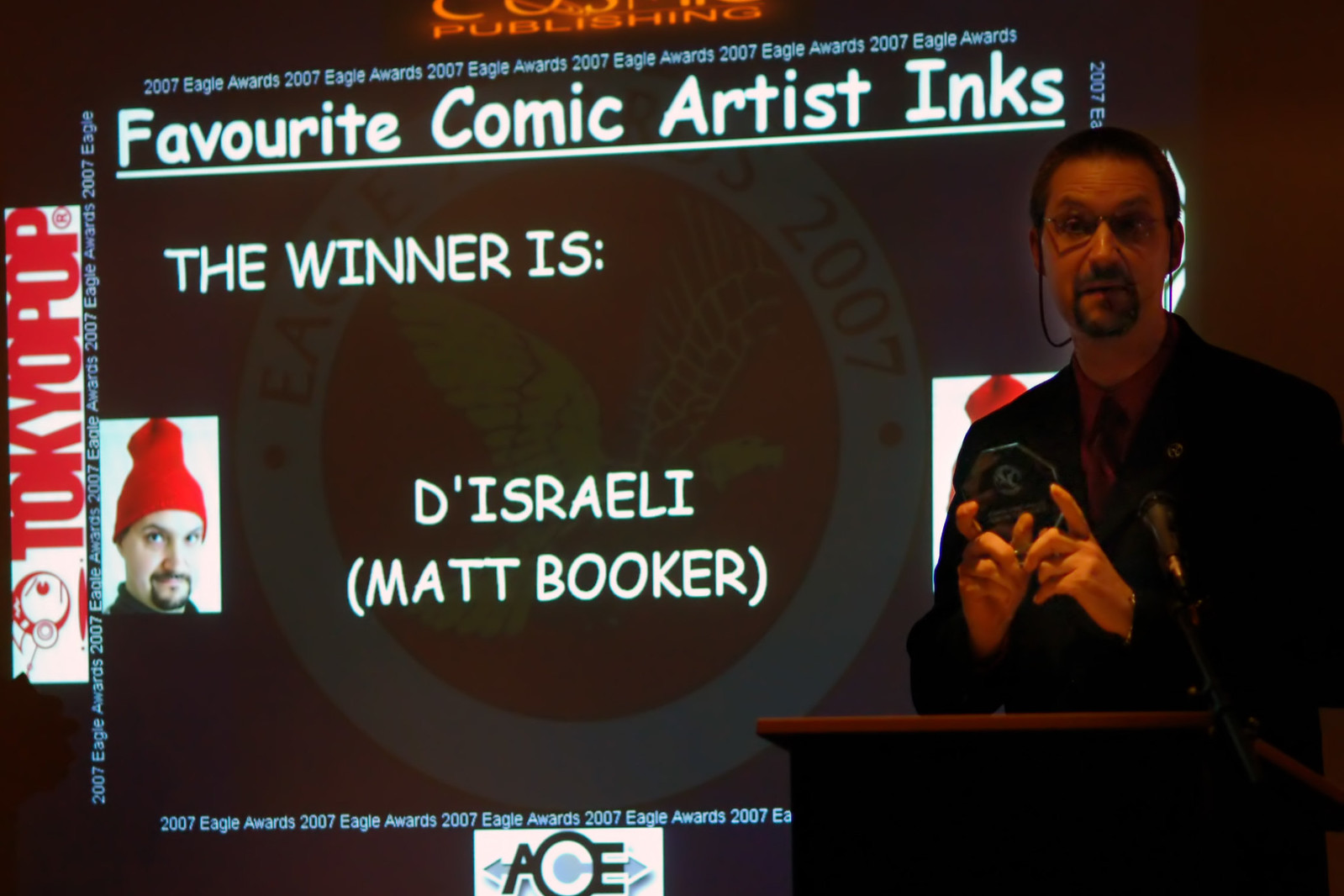In the image, a man stands at a brown podium on the right side, giving a presentation. He is wearing a black suit, a maroon shirt, and a red tie. The man, who is white with glasses connected by a small rope and a goatee, holds a small glass award in his hands. A microphone is in front of him as he looks towards the audience. Behind him on the left is a large projected screen, displaying the event information. The screen reads "2007 Eagle Awards" at the top and bottom, and in the center, it says, "Favorite Comic Artist Inks: The winner is the Israeli, Matt Booker." There is also a logo featuring an eagle in flight on a red background, encircled with the text "Eagle Awards 2007." On the far left of the screen, there is a small inset photograph of the award winner, Matt Booker. The screen is bordered by colorful logos, including "Tokyo Pop" with a space alien graphic on the left, and another logo reading "AOE" at the bottom. The setting appears to be indoors, likely during an award ceremony. The colors in the image are tan, light blue, orange, white, red, gray, brown, and black.